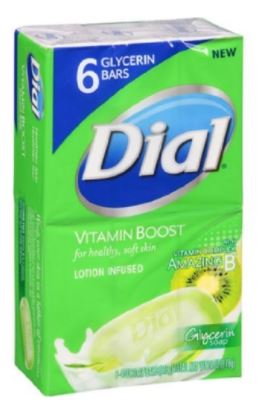The image features a pack of Dial Bar Soap, displayed against a white, frameless background. The packaging contains six glycerin soap bars and prominently features a green wrapper accented with blue highlights. In the top left corner of the package, there's a blue section indicating the quantity of soap bars. The central part of the package showcases a blue circle bordered in silver, with "DIAL" written in large, bold letters. Below this, in a light green area, it reads "Vitamin Boost for healthy, soft skin," followed by "Lotion infused." The image also depicts a bar of soap with drops of water beneath it, alongside a kiwi fruit slice positioned to the left and slightly behind the soap bar, showcasing the soap's partial side and the Dial branding. Additional details are present on the sides of the package but are not legible in this view.